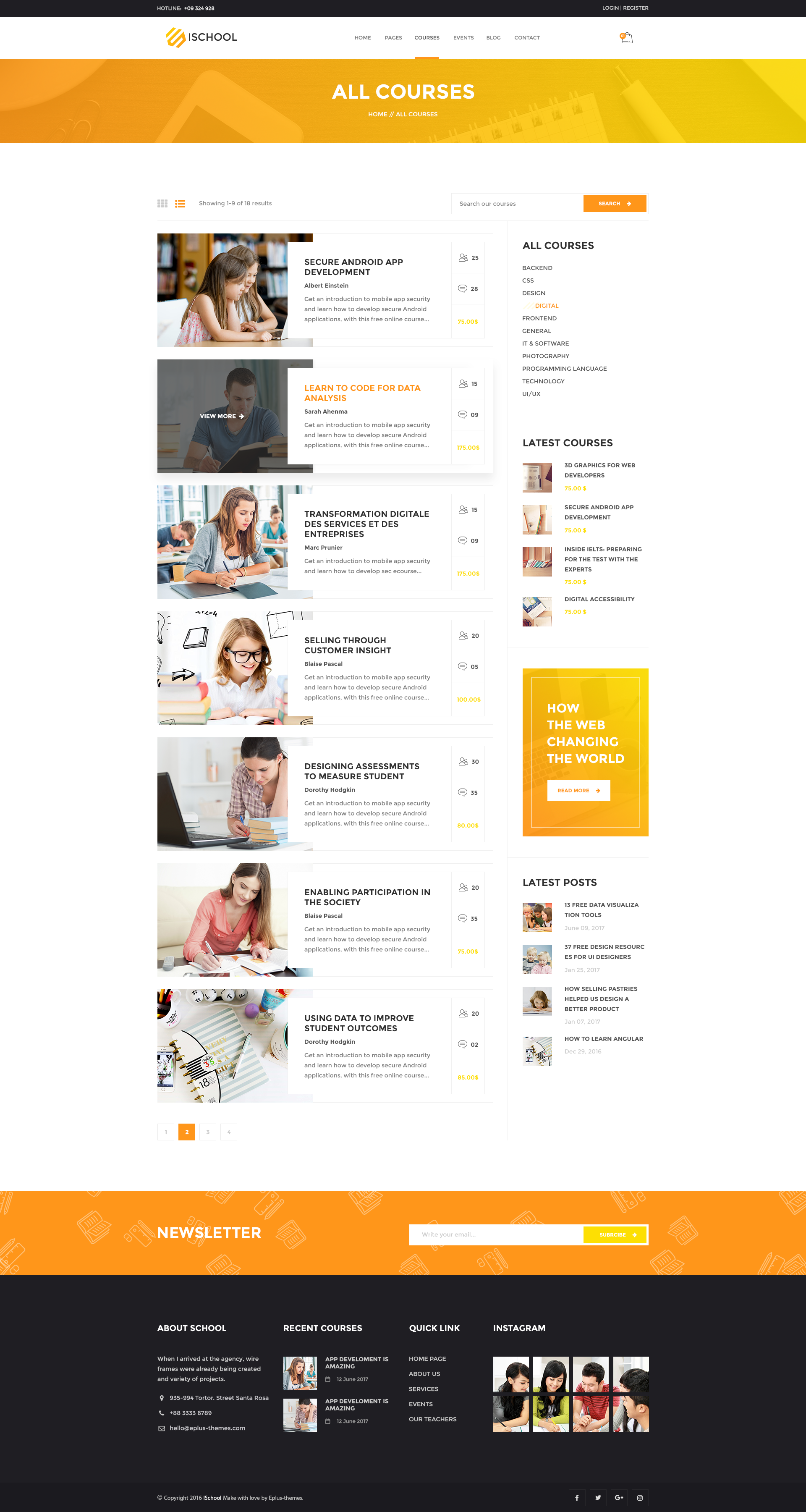This website page features a suite of business courses, prominently branded as "iSchool" at the top on a white background. Below the header, a vibrant yellow and orange banner declares "All Courses" in bold white text. Centered on the page are seven course links, each represented by a photograph and a descriptive title. 

1. The topmost image shows two young girls, accompanied by "Secure Android App Development" in black text over a white rectangle.
2. Below that, a man engrossed in reading books with the title "Learn to Code for Data Analysis."
3. Following is a young woman in a school setting, titled "Transformational Digital Services for Enterprises."
4. A little girl with books and glasses is featured under the title "Selling Through Customer Insight."
5. An image of a woman looking at a computer with books around her follows, titled "Designing Assessments to Measure Student Progress."
6. A young woman is next, her course titled "Enabling Participation in Society."
7. The final image in this section is of a notebook, labeled "Using Data to Improve Student Outcomes."

On the right side of the courses, "All Courses" is repeated, with various categories listed underneath. A prominent yellow rectangle asks, "How is the Web Changing the World?" Below this section are "Latest Posts," followed by an orange rectangle prompting visitors to sign up with their email for the newsletter. The very bottom of the page features a black background section with links for "About School," "Recent Courses," "Quick Links," and "Instagram."